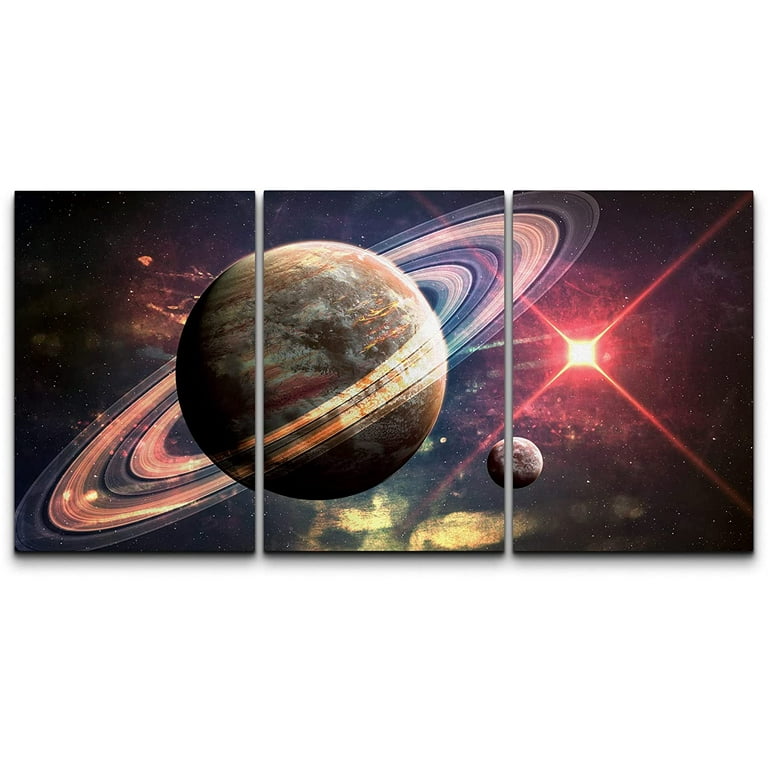This is a detailed three-panel canvas artwork featuring the majestic planet Saturn. The left panel showcases a portion of Saturn's planet body and part of its iconic rings, rendered in slate blue and white hues. The central panel displays the majority of Saturn, highlighting its gray and coppery surface, along with an expansive view of its rings wrapping around the planet. In the right panel, a distant shining star or sun emanates a warm amber and red glow, casting light across the scene in a striking X-shaped starburst pattern with four rays. A moon or celestial object orbits near the bottom of the right and middle panels, its presence partially divided by the thin separations between the sections of the artwork. The background is a dark, star-speckled expanse of the universe, adding depth and wonder to the galactic scene. Each segment of the triptych captures a unique aspect of the cosmic spectacle, blending together to form a cohesive and captivating portrayal of Saturn and its celestial surroundings.